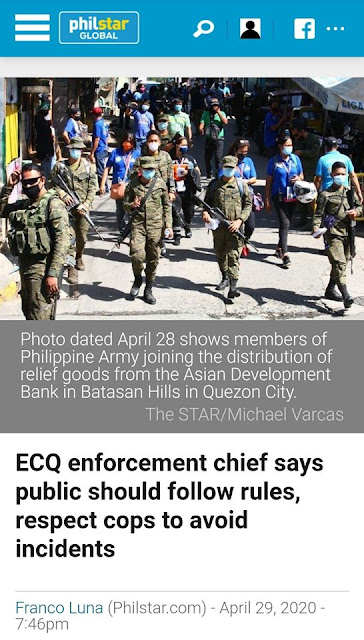The image is of a mobile phone displaying a website, specifically a newspaper article. At the top of the page, there is a light teal-colored rectangle featuring several icons and text. On the top left, three horizontal white bars signify the menu, followed by the text "Phil Star Global" enclosed within a thin white square. To the right, there are icons for search, profile (depicted as a black silhouette of a person on a white background), Facebook, and an ellipsis (three dots) for additional options.

Dominating the center of the webpage is a photograph depicting four military men, armed and clad in green camouflage uniforms. The soldier on the far left is equipped with a tactical vest loaded with magazine compartments. All four soldiers are facing forward, looking directly at the camera. In the backdrop, a crowd of civilians, some in blue shirts, can be seen.

Beneath this image is a light gray rectangle with the caption in white text: "Photo dated April 28 shows members of Philippine Army joining the distribution of relief goods from the Asian Development Bank in Batasan Hills in Quezon City." Attribution is given at the bottom right of this gray box, reading "The STAR / Michael Varcas."

At the very bottom of the webpage, against a white background, a black text headline reports: "ACQ Enforcement Chief says public should follow rules, respect cops to avoid incidents." Below this headline, the credit reads: "Franco Luna, Philstar.com," followed by a timestamp: "April 29, 2020, 7:46 PM."